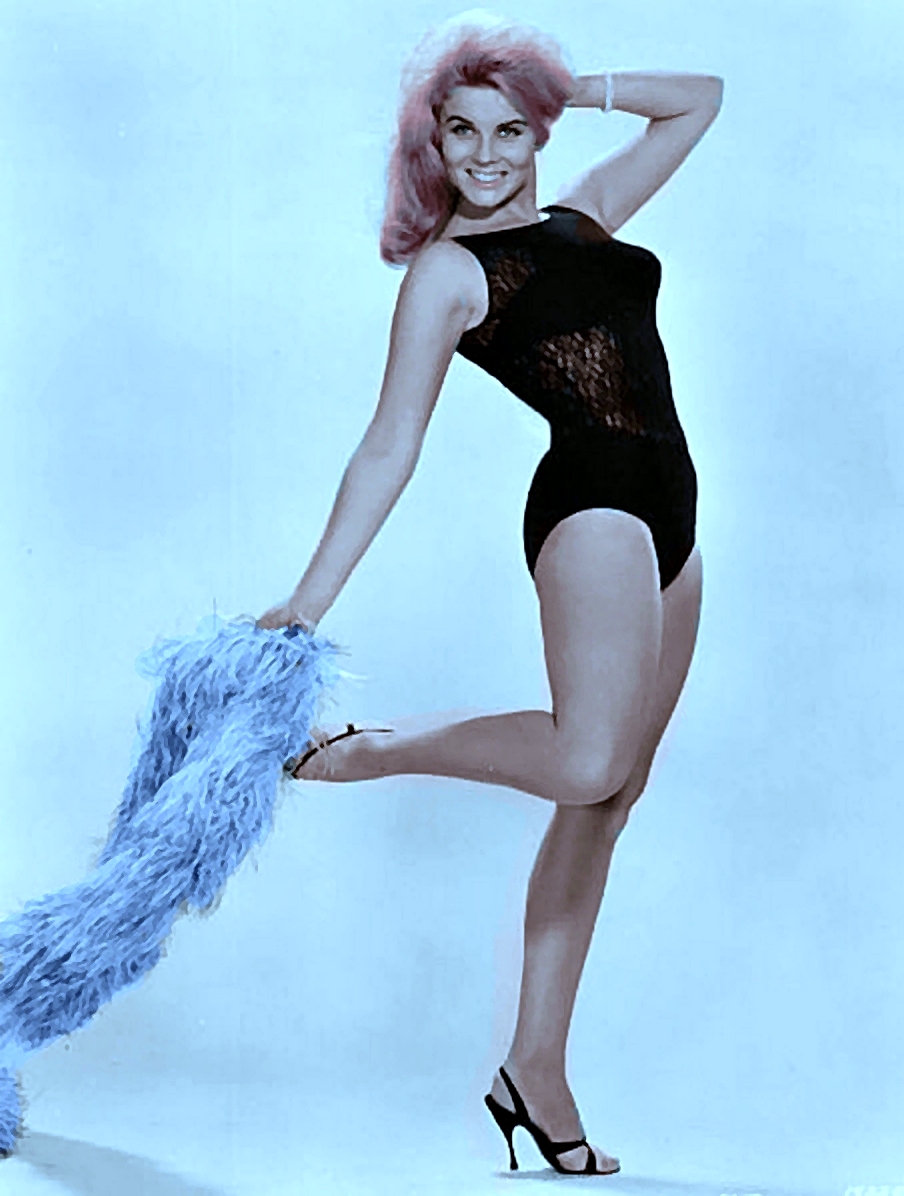This full-length, grainy-filtered photograph captures a strikingly beautiful woman posing like a model against a light blue background. She stands with her body facing towards the right, arching her back slightly while looking straight at the viewer. One leg is bent and lifted gracefully behind her, and she balances elegantly on black high heels. Her left hand is positioned behind her head at an angle, while her right hand delicately holds a long blue feather boa. Her black one-piece dress accentuates her poised figure, and her strawberry blonde hair adds a touch of elegance. The shadows under her heels subtly hint at the floor, completing this classic and stylish composition.